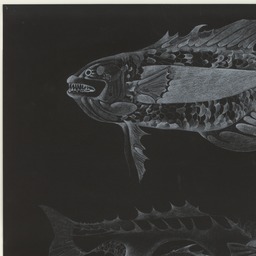In this compelling image, which exudes a dark and almost underwater ambiance, two fish are depicted in a stark black-and-white palette, reminiscent of an old, possibly centuries-old, illustration or an X-ray image. Both fish are rendered with an eerie level of detail that allows you to see their silhouettes as well as their internal structures, giving the image an X-ray-like effect. The upper fish, swimming to the left, is particularly detailed with visible facial features including round eyes, sharp, pointed teeth, and webbed fins. Its menacing appearance, with pronounced lips and hostile attributes, evokes a sense of danger, almost as if the fish could be a piranha. The lower fish, oriented to the right, is less defined but still showcases a skeletal interior and spiny fins. This fish appears murkier, with a grayish outline and darker interior, enhancing the abstract and treacherous feel of the scene. The entire composition, with its inverted negative effect and lack of colors, creates a haunting, alien-like portrayal of aquatic life.